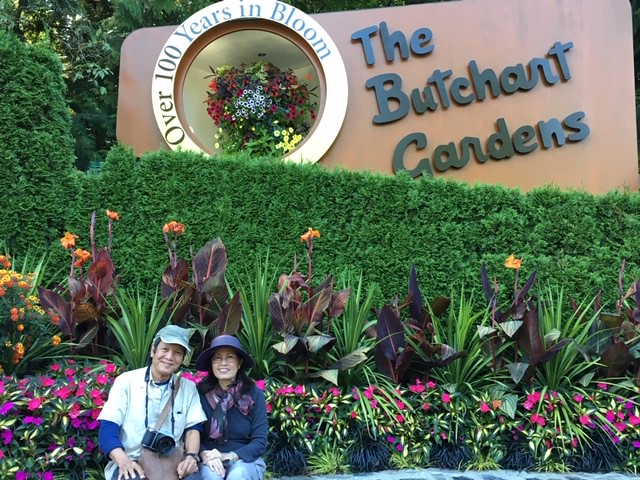The image captures an Asian couple sitting and posing in front of a vibrant garden display at The Butchart Gardens. The man, wearing a green hat, a white t-shirt over a blue long-sleeve shirt, and a watch, smiles faintly while an old-style camera hangs around his neck. Beside him, the woman wears a purple sun hat, glasses, a navy blue long-sleeve shirt, blue jeans, and a purple scarf. Behind them, a well-manicured array of pink and yellow flowers and lush green shrubs flourishes. A tan wall in the background features a sign in black script that reads, "The Butchart Gardens - Over 100 Years in Bloom," enclosed in a white circle.